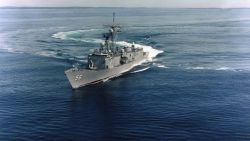This grainy, small, landscape photograph captures a modern gray warship gliding through an open, calm ocean. The image's bottom third shows dark blue, rippled water, transitioning to a lighter grayish-blue towards the horizon in the top half. The backdrop of the photograph features a thin strip of light gray sky. Central to the composition, the warship leaves a distinct S-shaped white wake in its path, indicating recent sharp maneuvers. The ship dominates the center of the frame and is characterized by its darker gray hull at the shadowed front, contrasting with a lighter gray side in the sun. Prominently, three rectangular gray structures rise from the deck—one near the front left, one centrally, and one at the rear right. From the central structure, a tall mast with a perpendicular component extends skyward. Additionally, three white cylinders are distributed across the tops of these rectangular forms, suggesting various technological equipment.